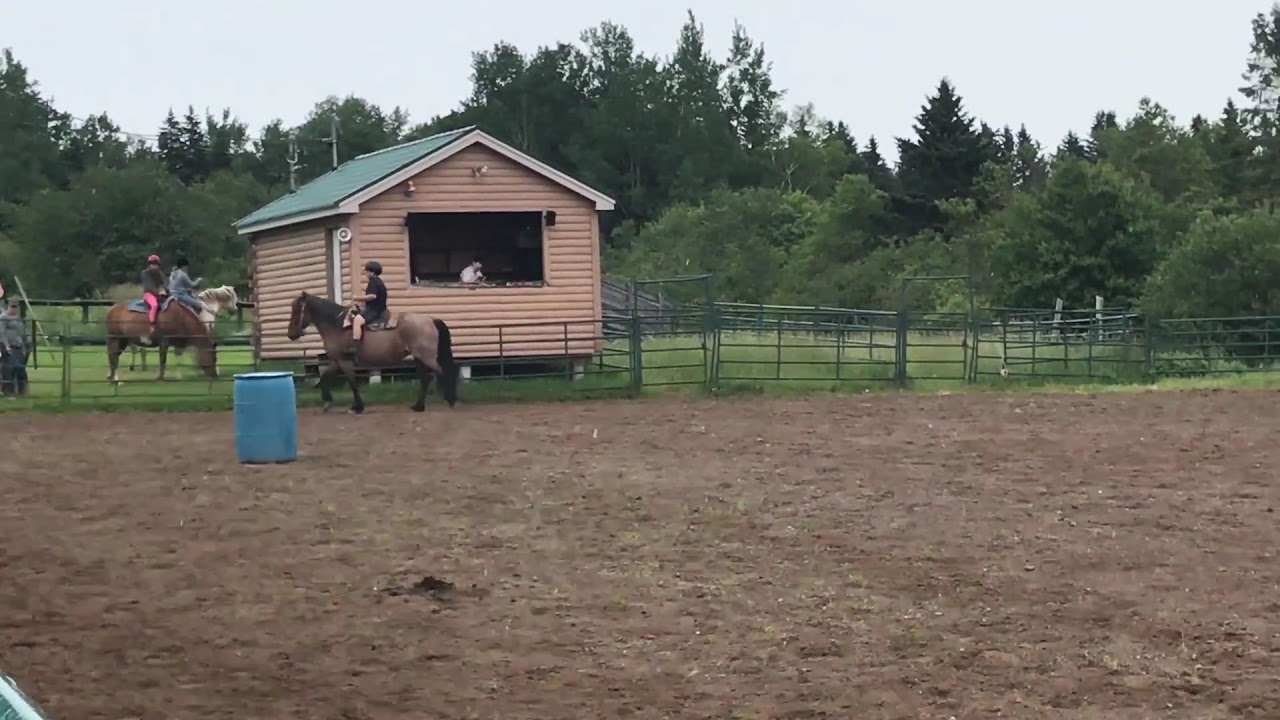The image is taken outdoors, showing a daytime scene that appears to be at an equestrian center, characterized by overcast skies and moderate weather suitable for t-shirts. In the foreground, we are standing in the middle of a dirt corral scattered with bits of chopped hay. A prominent blue rain barrel stands in the corral. Near the barrel, a young boy wearing a black helmet, black shirt, shorts, dark socks, and dark shoes is riding a brown pony with a black mane and tail. 

Behind him, a green metal fence runs along the back of the corral. Just beyond this fence, there is a small log cabin or shed with a green slanted roof. To the left of the cabin, two people are on horses—a brown horse and a white horse. One of the riders is wearing bright pink pants and a pink helmet.

The background is filled with tall green grass, rows of trees, and bushes, enhancing the natural, outdoor setting of the scene. The overall atmosphere suggests a peaceful day in a rural area dedicated to horse riding activities.